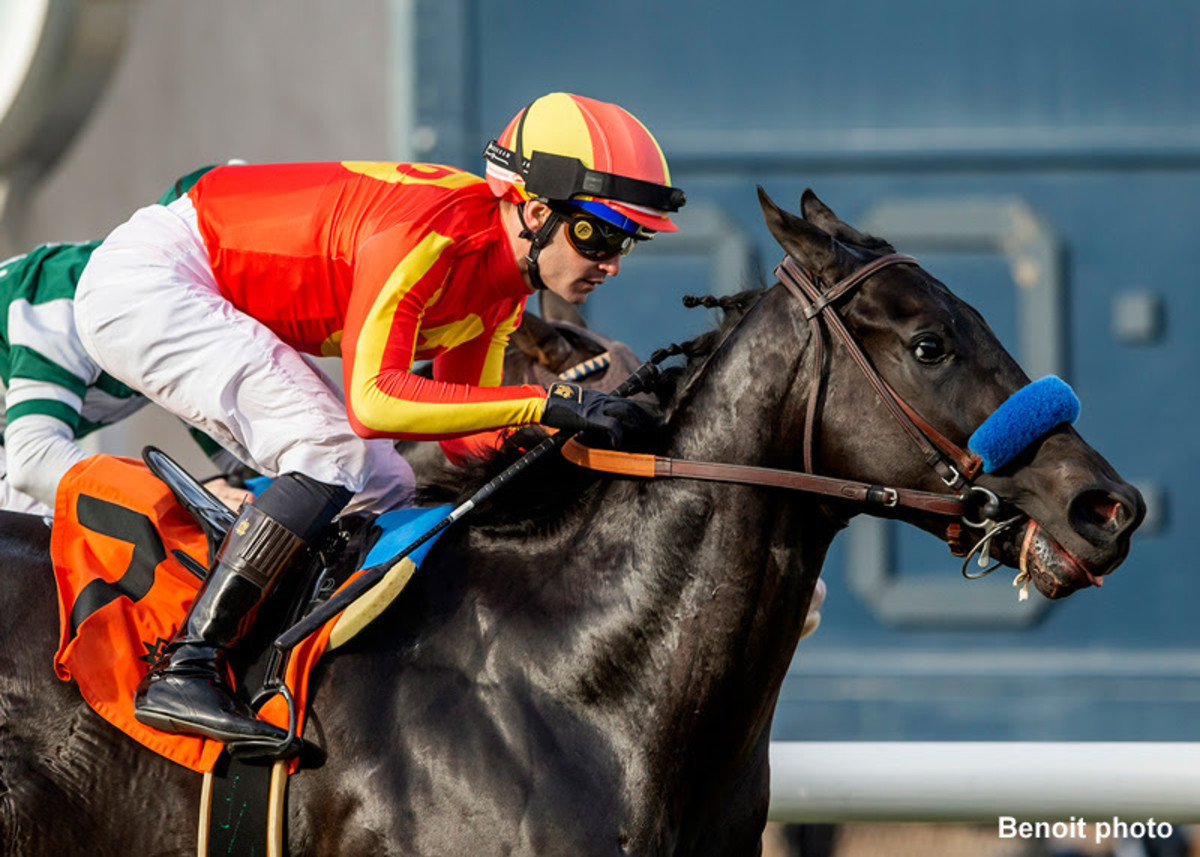The photograph captures an intense moment just before a horse race. At the center, a jockey rides a sleek black horse. The horse is fitted with a brown leather bit in its mouth, connected to brown straps, one of which features a padded blue covering along the nose. The jockey, a small man, is clad in a striking red and yellow striped shirt, with matching helmet, white racing pants, and tall black boots. He is crouched over in a squatted position, half-standing in the stirrups, clutching both the reins and a riding crop in his right hand. The saddle beneath him is a vibrant mix of blue, yellow, orange, and black. Behind him, another jockey in a green and white uniform is partially visible, riding a light brown horse. The background transitions from a grayish hue on the left to various shades of blue on the right, including a distinctive white line that bears the text "Benoit Photo" in white.